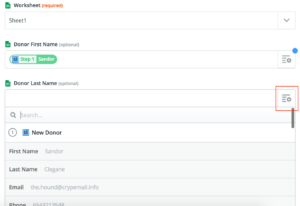This image is a blurred and out-of-focus cropped screenshot of a worksheet generator interface, likely from Google Docs. The background of the interface is white. In the upper left corner, there is a green document logo followed by the word "Worksheet" in black text. Directly to the right of "Worksheet," there is a red "Required" label. Below this header, there's a drop-down box with "Sheet 1" selected.

Further down, another header features a green document icon followed by the text "Donor First Name" labeled as optional. Under this, there are several green options with a document icon to the right, each with a blue dot in the top right corner, indicating that you can add new documents or edit existing names. Below this section, there is an area labeled "Donor Last Name" accompanied by a text box. Beside this, there is an edit button, which shows a document icon with a plus symbol, edited with a red box to highlight it as the button to press for editing. When this button is maximized, a search bar appears below. Finally, the section labeled "New Donor" is visible, followed by contact card information.